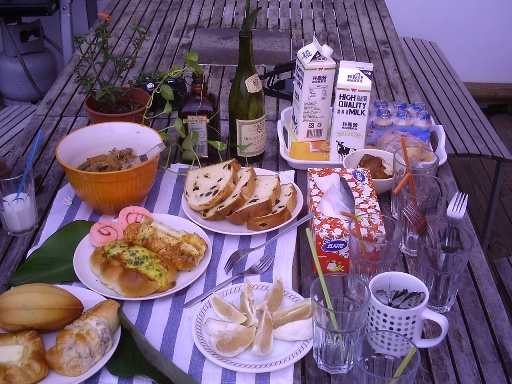This detailed photograph depicts an outdoor picnic or breakfast scene on a worn, weathered wooden picnic table with matching stools or benches made from the same wood. The table’s thin vertical slats of wood are closely set together. Center and toward the left of the image there's a variety of food spread out on the table. A white plate with cut-up oranges is visible next to another plate featuring four slices of chocolate raisin bread. Several pastries are scattered around, including one that resembles a cheese danish and another shaped like a football.

In the lower left-hand corner, there's a white and blue striped cloth under a white plate of pastries. An orange bowl with white inside and some tongs is seen nearby. Various utensils are distributed around—forks, spoons, and glasses with blue and green straws. A cup holds spoons, and another glass holds forks.

Among the items, there’s also a red Kleenex box, a couple of jugs labeled "high-quality milk," a six-pack of bottled water, and a green bottle of wine. Additionally, there's an unidentified bottle, possibly liqueur, two glasses filled halfway with milk and straws, and a cup with more utensils. A flowering plant in a pot, with some vines trailing, serves as a decorative element on one side. The table recedes away from the viewer, showing an empty section at the far end. The photograph is rectangular, about three inches tall and four inches wide, capturing a serene yet lively outdoor dining setup.